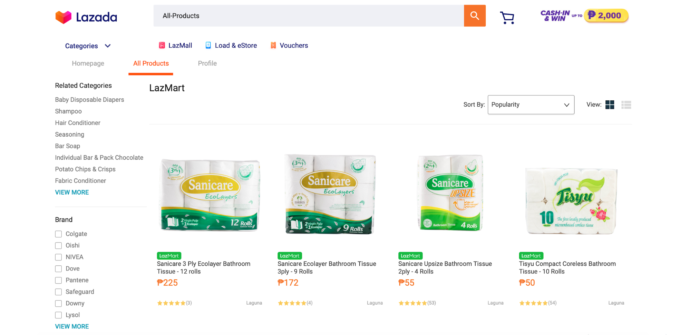On the Lazoda.com homepage, the search bar is prominently featured alongside a shopping cart and the "Cash-in-and-win" banner, advertising a chance to win P2000. Multiple options are available, including 'LASMAIL', 'Load and Visit', and 'eStore'. Shoppers can access vouchers, view all products, and navigate to their profile from the main page. The categories section offers a range of products such as baby items, including disposable diapers, as well as personal care products like shampoo, hair conditioner, bar soap, and fabric conditioner. Snacks such as potato chips, crisps, and a variety of chocolates are also listed.

The site features popular brands like Colgate, Oishi, Nivea, Dove, Pantene, Safeguard, Downey, and Lysol. Under the bathroom tissue category, specific products are highlighted such as Sanicare 3-ply eco-player bathroom tissue (12 rolls for P225), Sanicare eco-layer bathroom tissue (3-ply, 9 rolls for P172), Sanicare up-size bathroom tissue (2-ply, 4 rolls for P55), and Tissue Compact Coreless bathroom tissue (10 rolls for P50). A side comment humorously notes the finger-poke vulnerability of the compact coreless bathroom tissue.